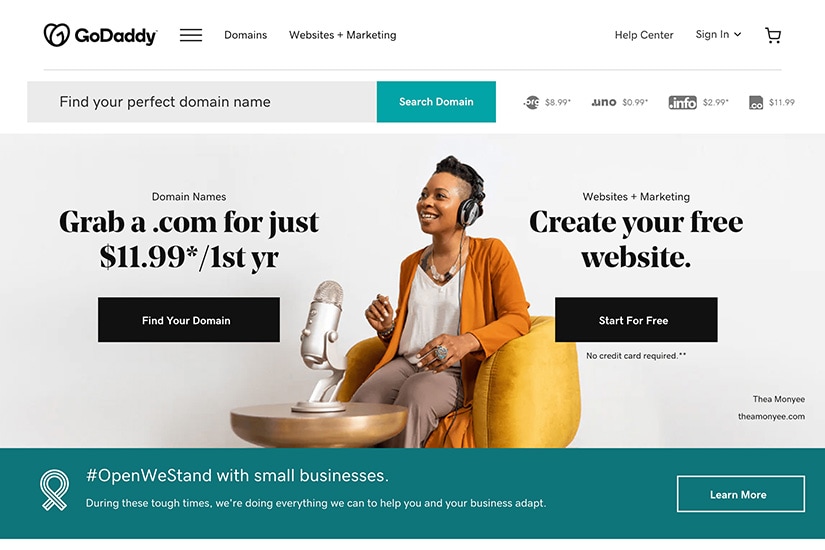The image showcases a landing page for GoDaddy.com, prominently featuring the GoDaddy logo in the top left corner. The website's header includes navigational links to "Domains," "Websites and Marketing," "Help Center," a "Sign In" option, and a shopping cart. Below the header is a search bar prompting users to "Find your perfect domain name" and a button labeled "Search Domain."

Central to the page is a vibrant image of a black woman seated on a chair, equipped with headphones and speaking into a podcast microphone, suggesting she is actively involved in podcasting. Adjacent to this image, on the left, there is a promotional message: "Domain Names - Grabby.com for just $11.99 for the first year," along with a call-to-action button labeled "Find Your Domain."

To the right of the woman’s image, the focus shifts to website creation with the text "Websites and Marketing - Create your free website" accompanied by a "Start for Free" button.

At the bottom of the landing page, a green footer contains a supportive message: "Open We Stand with Small Businesses. During these tough times, we are doing everything we can to help you and your business adapt." This section also includes a "Learn More" button for additional information.